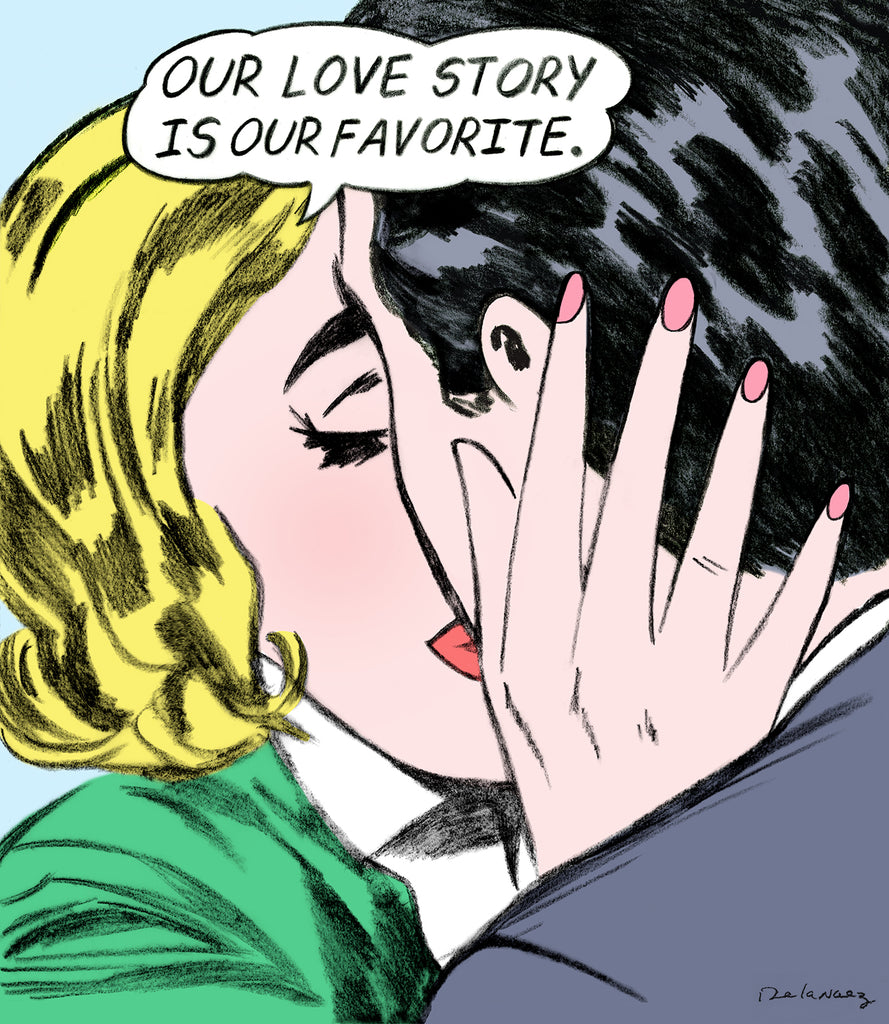The image is a colorful drawing reminiscent of an old comic book, depicting a heartfelt moment between two people kissing at its center. The woman, positioned on the left, has blonde hair, red lipstick, black-outlined eyelashes, and pink fingernails. She wears a light green jacket over a white blouse, and her right hand gently touches the man's face. The man, seen from the back on the right, has black hair and wears what appears to be a gray suit jacket. Above them, a dialogue bubble with a cloud-like shape contains the phrase, "Our love story is our favorite." In the bottom right corner, there's a signature from the artist. The overall style of the image is simple and evocative, typical of a classic comic strip.